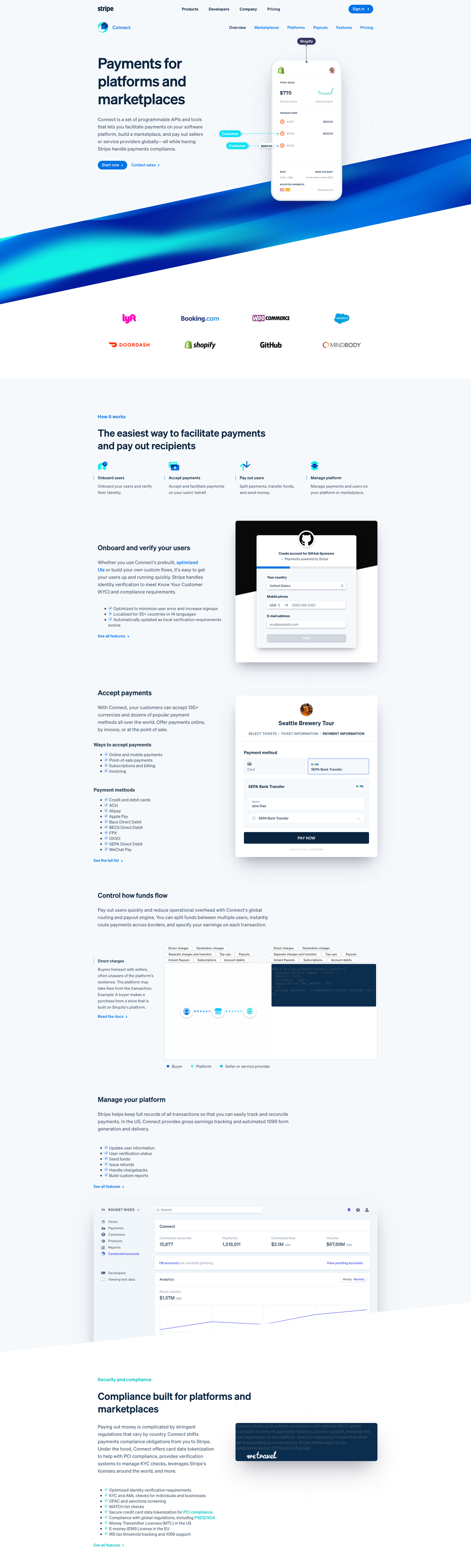The image depicts a web page interface predominantly featuring a very light blue background, almost white in its hue. Approximately 10-15% down from the top, the page has a distinctive blue bar extending horizontally across the width, angled slightly upward. This blue bar, occupying about 5% of the image, showcases a combination of light blue, dark blue, and medium blue wave patterns, creating a visually dynamic element. In the upper left corner above this bar, there is some indistinct text, likely indicating the page's header or section title. Surrounding this area are additional small text elements, the details of which remain unclear due to their small size and blurriness. Embedded within the interface are various clickable blue buttons that presumably navigate to different sections or options of the web page. Below the blue bar, the main content area appears to be displaying a specific page with extensive text information, accompanied by contextual options or interactive elements related to the content being described.